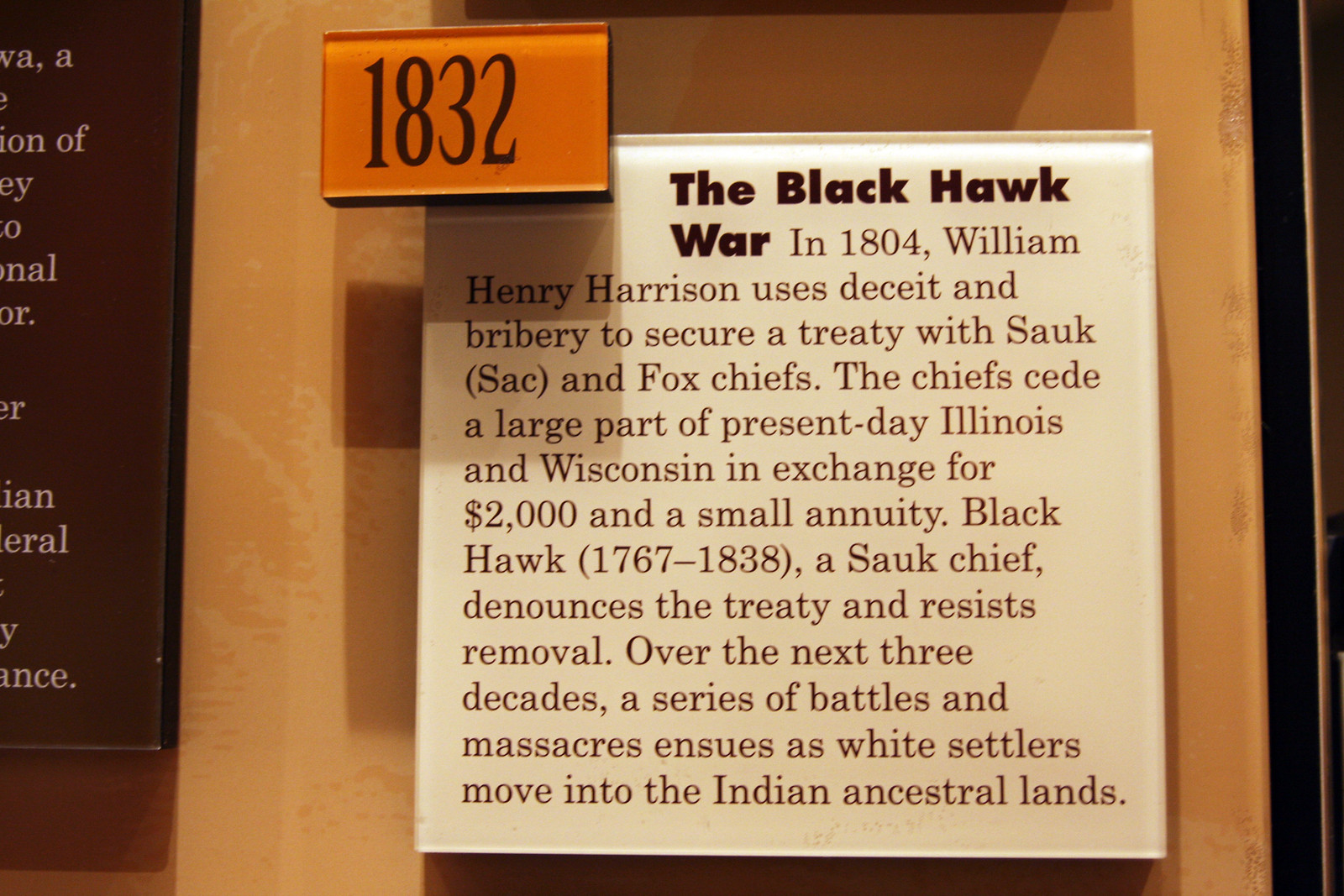The image depicts a historical display sign, prominently featured on a light wood wall. At the top left, there is a small orange plaque inscribed with "1832" in black letters. Below this, the main square sign has a white background with black text. The title, "The Black Hawk War," is in bold. The detailed text explains that in 1804, William Henry Harrison employed deceit and bribery to secure a treaty with the Sauk (SAC) and Fox chiefs. These chiefs ceded a large part of present-day Illinois and Wisconsin in exchange for $2,000 and a small annuity. Black Hawk, a Sauk chief born in 1767 and living until 1838, denounced the treaty and resisted removal. Over the next three decades, a series of battles and massacres erupted as white settlers encroached upon the Indian ancestral lands. The sign sits partially surrounded by other signs in the display area.